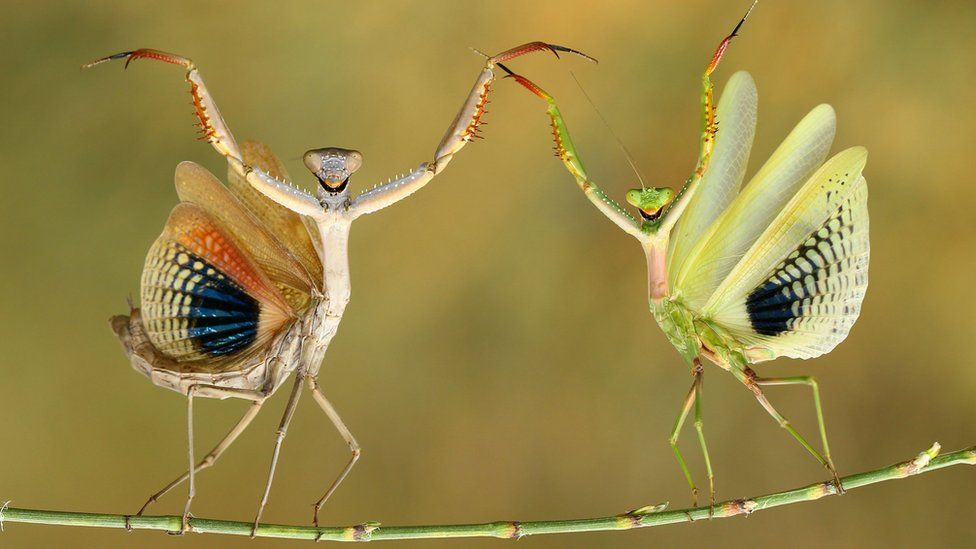The image depicts a detailed and vibrant scene of two stylized praying mantises perched on a slender green twig that stretches horizontally from the left to the right of the composition. The background features a blurred amalgamation of greens, yellows, and browns, accentuating the focus on the two insects.

On the right side, a green-bodied mantis poses with its arms raised in a triumphant Y-shape. This mantis has a green face with light green eyes, and its limbs are notably colorful, featuring green forearms that transition into red-tipped purple accents. Its wings are prominently white with a gradient of dark blue and blue specks, and yellow edging towards the tips.

The mantis on the left stands in a mirrored pose with its arms similarly raised. Its body is brown with hints of white, and it exhibits wings that are a composite of brown, dark blue, and vibrant patterns including red, yellow, and blue speckles. It faces the audience, displaying a sense of interaction as its eyes and stance suggest a ready engagement with the viewer.

The twig they stand on is nuanced with green, yellow, and brown patches, adding to the lifelike quality of the scene, even as it unmistakably blends elements of fantasy through the vivid colors and attributes of the mantises. Both mantises appear to be stationary, seemingly engaged in a synchronized display or dance, their positions giving them an almost joyful and animated character.